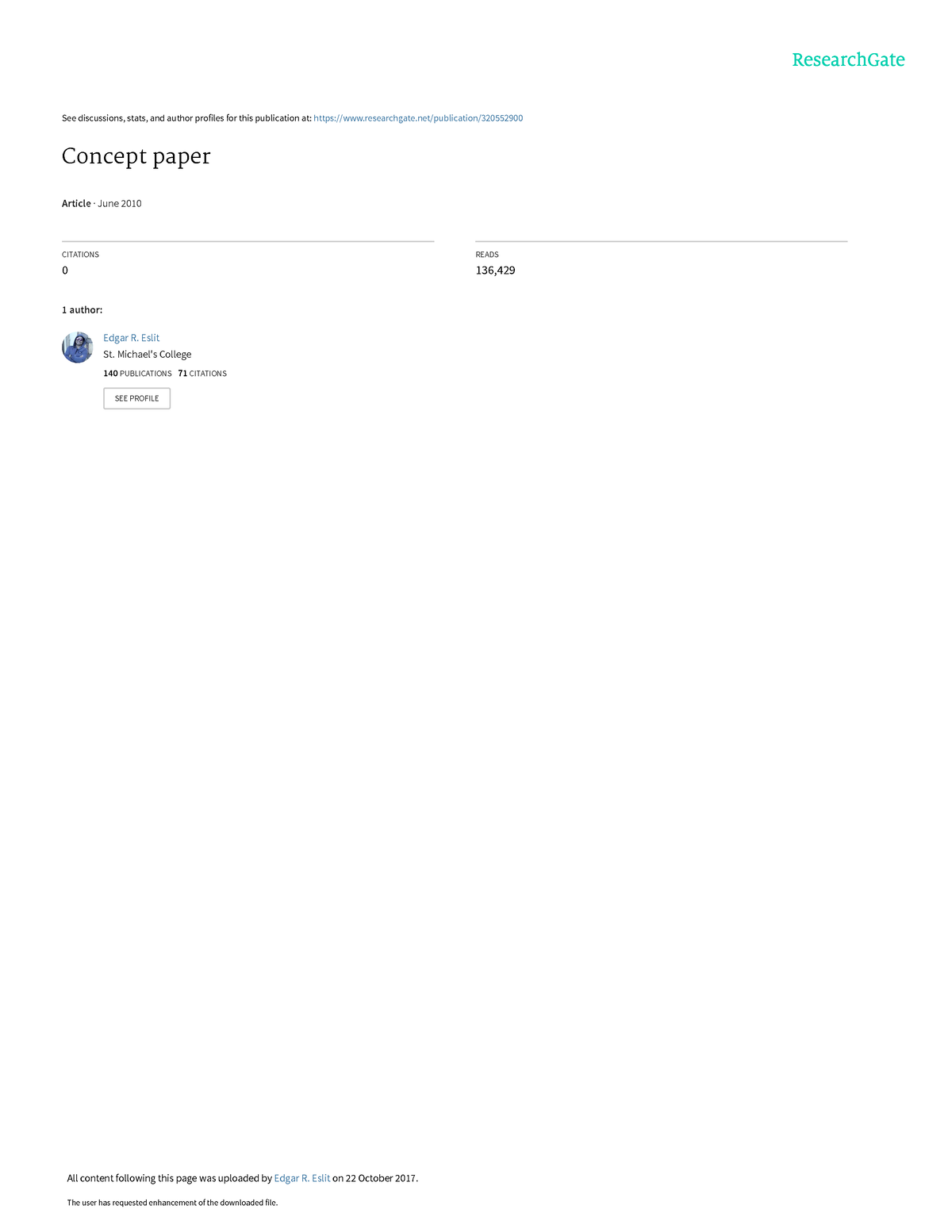The image depicts a white background with various textual elements displayed prominently. At the top right corner, the word "ResearchGate" is written in green. On the left side, there is a block of text that reads: "Seed Discussions, Stat and Autoprofile for this publication," followed by a blue URL: "researchgate.net/publication/32055202900."

Below this text on the left, there's additional information stating: "Concept paper, article June 2010. Citation: 0." Alongside on the right, the image shows: "Reads: 136,429," indicating the number of times the publication has been read.

Further to the left, it mentions: "One author," accompanied by a profile picture of the author, Edgar R. Eslit, who is depicted wearing a blue suit. The name "Edgar R. Eslit" appears in blue text next to the black text that mentions his affiliation with "St. Michael's College - Art and Food." Below this, a line reads: "Publication: 71, Citation."

At the bottom left of the image, there's a disclaimer in black text: "All content following this page was uploaded by Edgar R. Eslit on 22 October 2017. This user has requested enhancement of the downloading file."

Overall, the image is primarily informational, delineating specific details about a publication on ResearchGate, including author information, publication metrics, and a disclaimer regarding the content upload date.